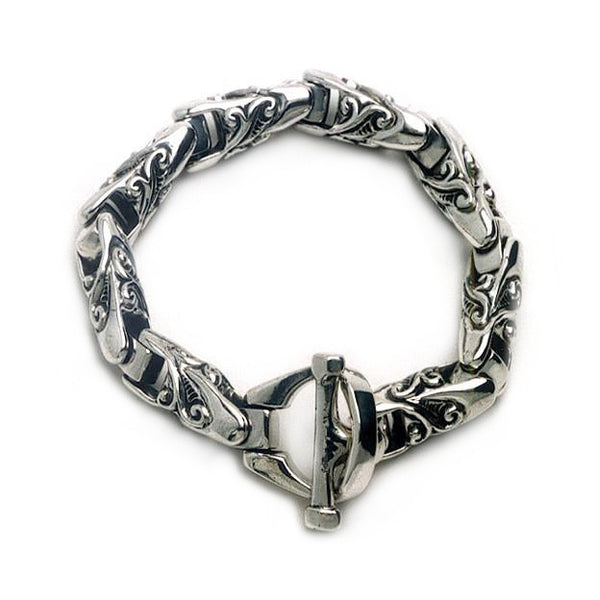The image features an intricate, antique-looking silver bracelet. This finely detailed piece is composed of multiple linked segments, each displaying a design reminiscent of a tulip, with a gentle upward curving horn and two curved leaves curling back toward the stalk. The bracelet's clasp operates with a barbell mechanism that passes through a circular loop, securing it in place when laid flat. The bracelet is currently fastened, giving the appearance of being ready for wear. The entire bracelet exhibits a consistent silver color, enhancing its elegant and sophisticated aesthetic.